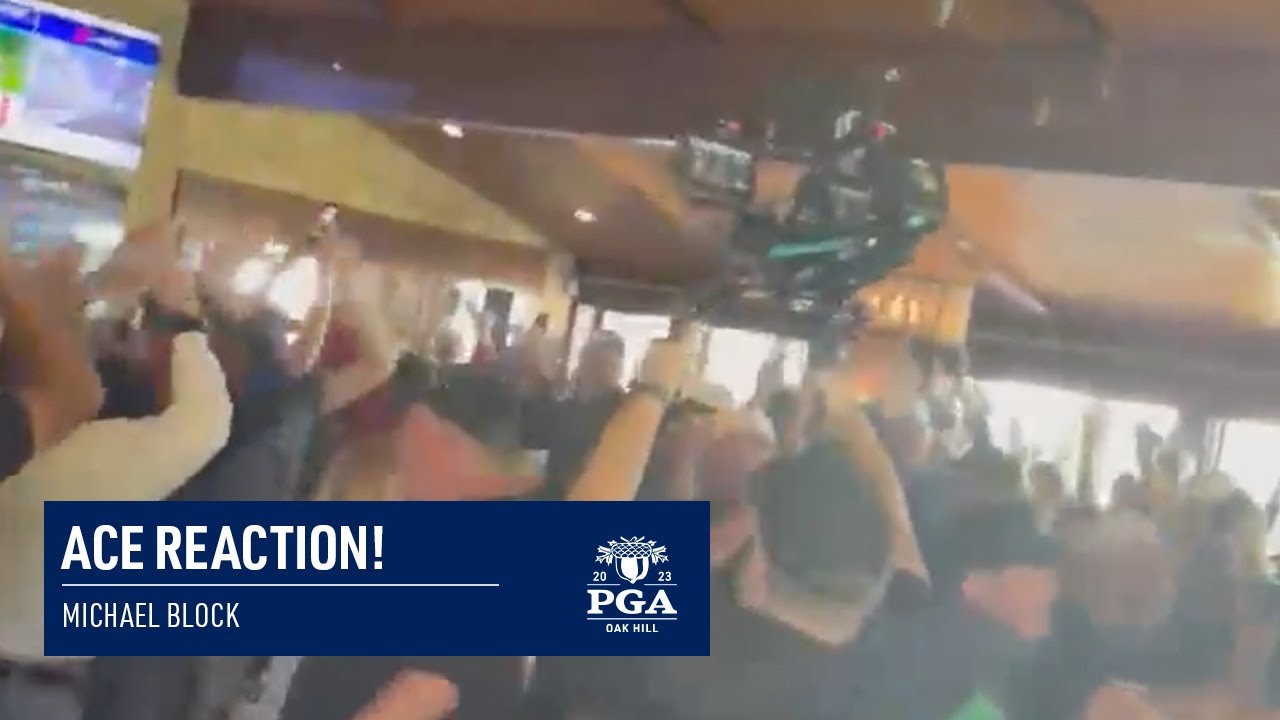The horizontally aligned, somewhat fuzzy image appears to be a photograph or a digitally rendered painting capturing a crowded indoor scene, possibly inside a club or hotel setting. The focal point is an enthusiastic crowd that stretches diagonally across the image from top left to bottom right, with many people raising their arms, some with fists clenched in excitement. Notably, on the far left, a person in a white long-sleeved shirt stands with their back to the viewer.

In the background, there are two rows of nearly square windows framed in dark color, extending diagonally downwards from left to right, alongside a ceiling adorned with lights and paneling in shades of brown and tan. Above the windows, a possible TV screen displays indistinct images in green and pink hues, bordered by a blue banner with a logo, reinforcing the environment as a lively, possibly sports-centered venue. 

The bottom left corner of the image prominently features a blue banner about 3 by 10 centimeters in size. On this banner, text in white capital letters reads "ACE REACTION," and beneath it, a smaller horizontal line leads to the name "Michael Block." The right side of the banner includes a white acorn icon flanked by leaves, with the year "2023" split around the acorn. Below that, another horizontal line bisects the word "PGA," followed by a final line stating "Oak Hill" in the smallest text. The combined visual and textual elements hint at a celebration or event likely related to the PGA at Oak Hill, complete with festive crowd reactions and a professional setting.